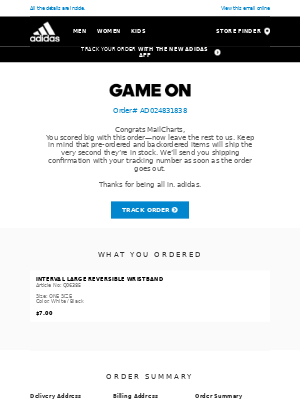The order summary page from Adidas prominently features the Adidas logo at the top in white lettering against a black background. The navigation options include "Men," "Women," "Kids," and to the right, a "Store Finder" icon represented by a small circular symbol with a black dot. There's also a message that reads, "Track your order with the new Adidas app."

Beneath this section, on a white background, an eye-catching bold message in capital black letters states, "GAME ON." Below this, the order number AD024831838 is listed. The following message, in black letters, congratulates the customer, saying, "Congrats, Mall Charts! You scored big with this order, now leave the rest up to us. Keep in mind that pre-ordered and back-ordered items will ship the very second they're in stock. We'll send you shipping confirmation with your tracking number as soon as the order goes out. Thanks for being all in Adidas."

A blue rectangle button with white lettering invites the customer to "Track Order."

Further down, on a light greyish-white background, the section titled "What You Ordered" is in black lettering, followed by a detailed list of the items ordered. The details of each item include the product description, which is "Integral Large Reversible Wristband," an article number, the color, and the price of $7.

Finally, on a white background, the order summary concludes with sections for "Delivery Address," "Billing Address," and a recap of the "Order Summary," all written in black.